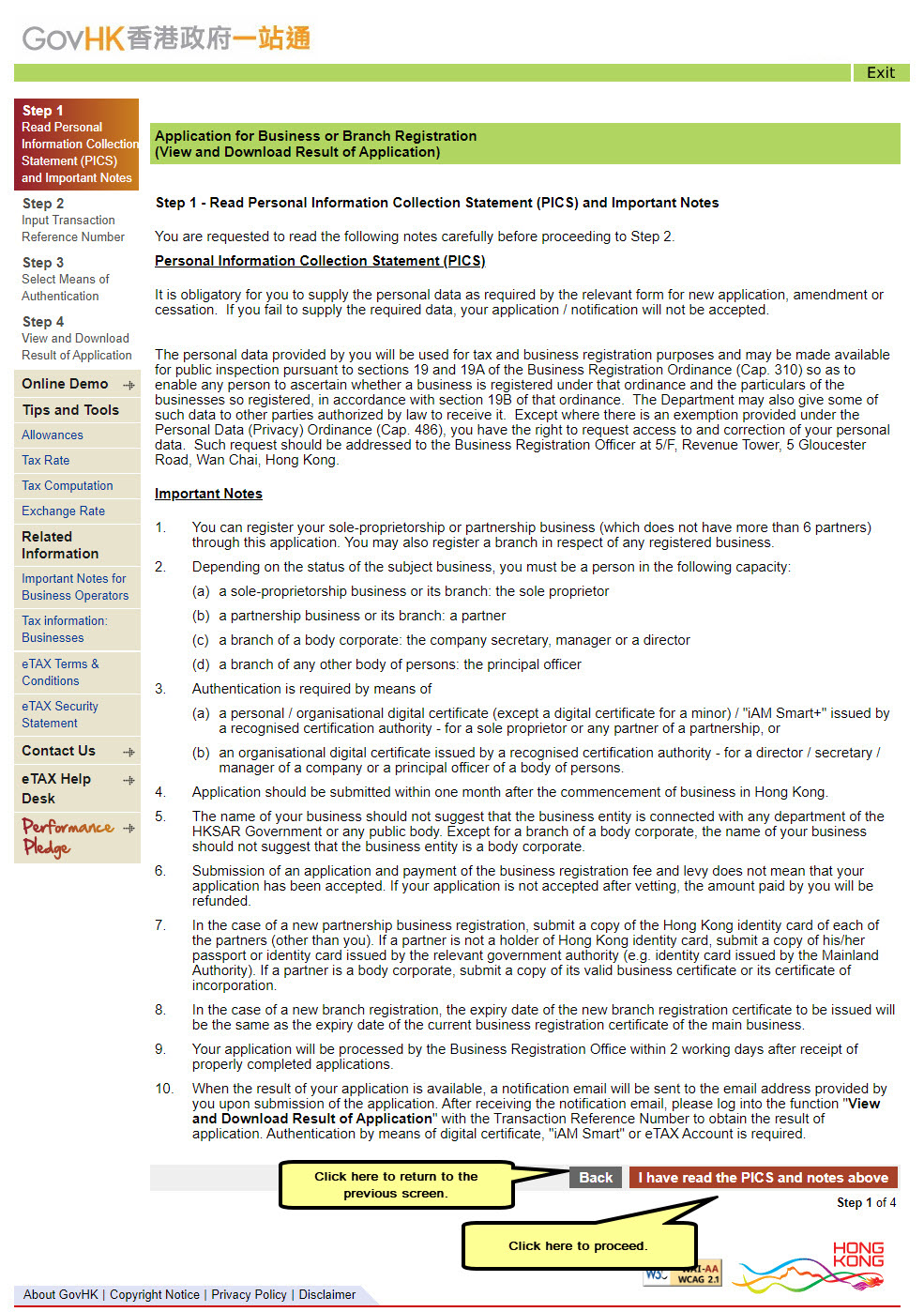This image, sourced from a website, presents an online form titled "Application for Business or Branch Registration." The header, adorned with elegant Asian text, adds a culturally rich aesthetic, though the specifics of the script are not readable. Moving down, the page instructs users to "View Download Results of Application." 

Step one is prominently highlighted, instructing users to "Read Personal Information Collection Statement (PICS) and Important Notes." Below this heading, a detailed text block offers important notes and guidelines, numbered sequentially from one to ten. 

At the bottom of the instructions, various informative speech bubbles point to key areas of the form. There are two prominent buttons: a "Back" button labeled "Click here to return to the previous screen" and another that reads "I have read the PICS and notes above," encouraging users to click to proceed.

On the left side of the image, a vertical series of steps is displayed. Step one is marked in a red box, while steps two, three, and four follow in a connected white box sequence. A tan box containing additional information is positioned at the bottom of this column, completing the detailed step-by-step instructions for the registration process.